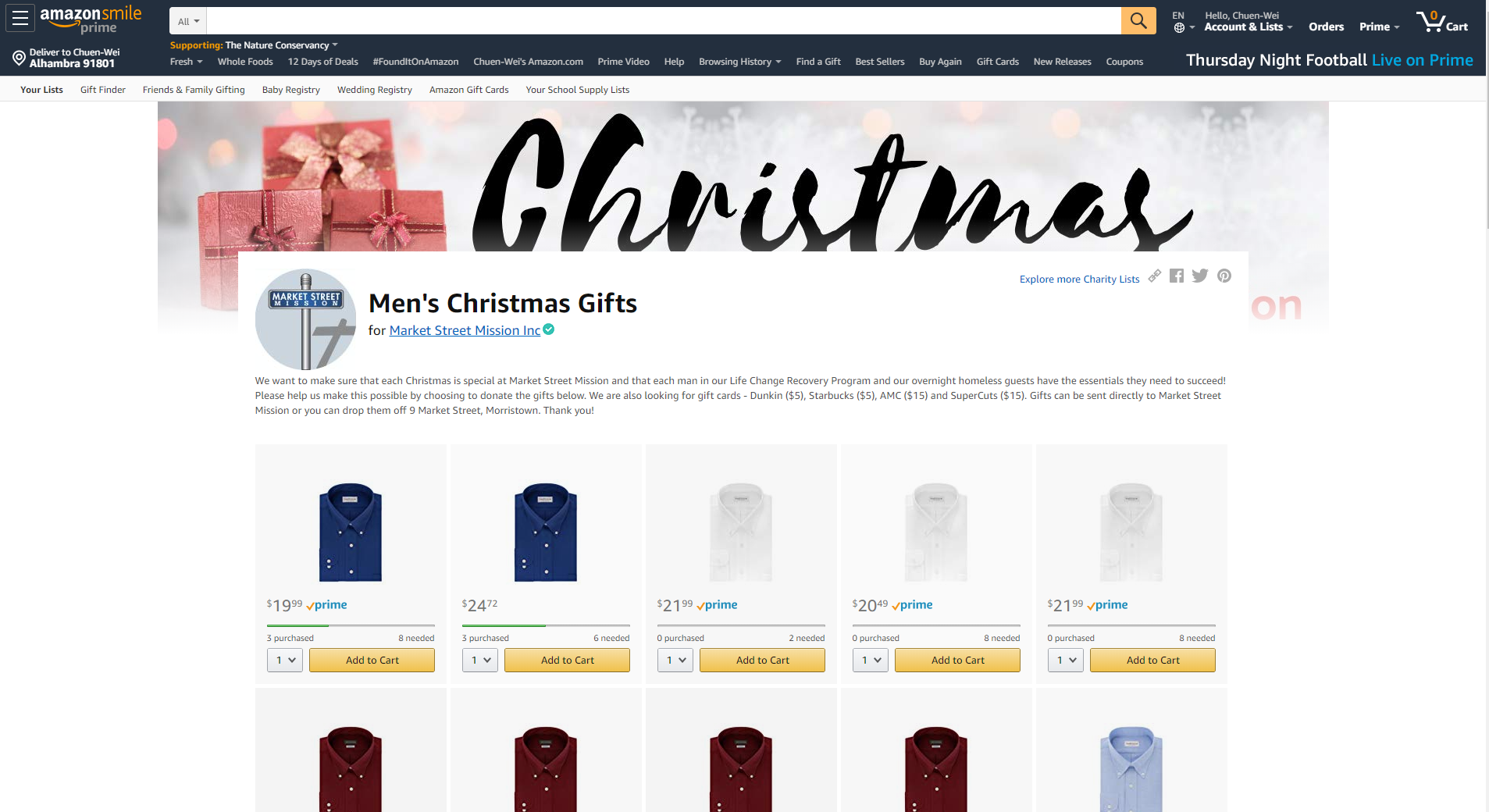The image is a screenshot from an individual's Amazon Smile account. At the top of the page, it is noted that the user is supporting the Nature Conservancy through their purchases. The banner also indicates that the user is logged in as "Chen Wee" and highlights an advertisement for Thursday Night Football Live on Prime. The cart icon at the top displays zero items.

The main content of the page is focused on men's Christmas gifts, specifically showcasing a selection of button-down shirts. There are two rows of shirts displayed neatly. The top row features five shirts: two navy blue shirts on the left followed by three white shirts. The prices and Prime eligibility for these shirts are as follows:
- First navy shirt: $19.99, Prime-eligible
- Second navy shirt: $24.72
- First white shirt: $21.99, Prime-eligible
- Second white shirt: $20.99, Prime-eligible
- Third white shirt: $21.99, Prime-eligible

The bottom row features four burgundy shirts and one blue shirt on the far right. However, the prices and Prime eligibility details for these shirts are not visible in the screenshot.